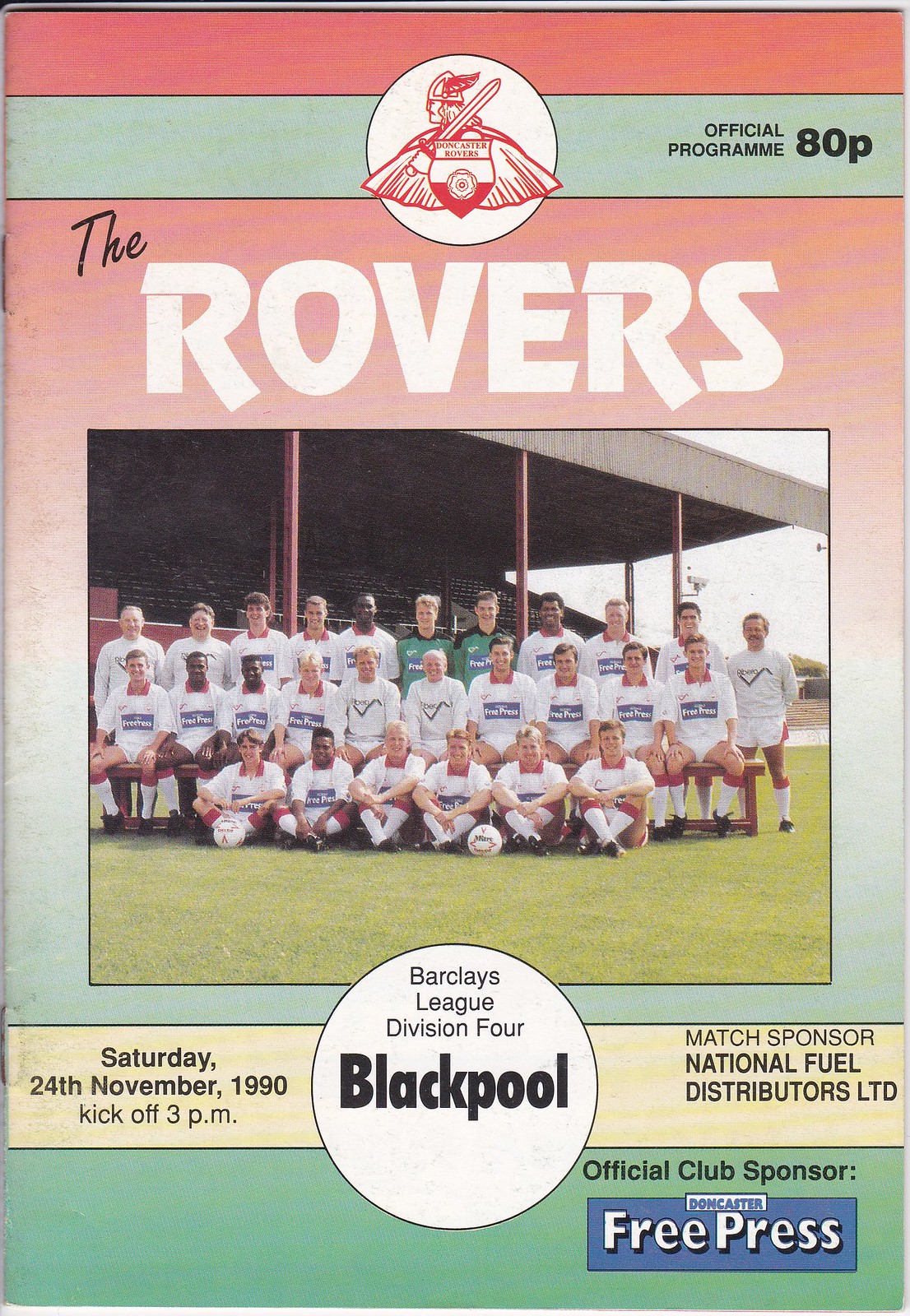This is a photograph of an old soccer team program, featuring vibrant colors transitioning from red to yellow to soft green on the cover. Dominating the top portion is the team's logo, a white circle depicting a sword, shield, and a Viking helmet, with the title "Official Program ADP" adjacent to it in black letters on a gray strip. Below the logo, the team's name "The Rovers" is prominently displayed in black and white letters against the variegated background.

A group photo of the men's soccer team, positioned centrally on the cover, showcases the players donning predominantly white jerseys, although a few are clad in green and black kits. They are posed on a green soccer field with the stadium bleachers looming in the background, complemented by a couple of white soccer balls with black and red writing.

Beneath the team photo, a white strip cutting across the green background lists the match details: "Saturday, 24th, November, 1990, kickoff, 3 p.m.” The text further identifies the event as part of the “Barclays League Division IV Blackpool," with "National Fuel Distributors Limited" credited as the match sponsor. At the very bottom, the "Official Club Sponsor" is acknowledged as "Doncaster Free Press" on a combination of white and blue backgrounds with alternating text colors.